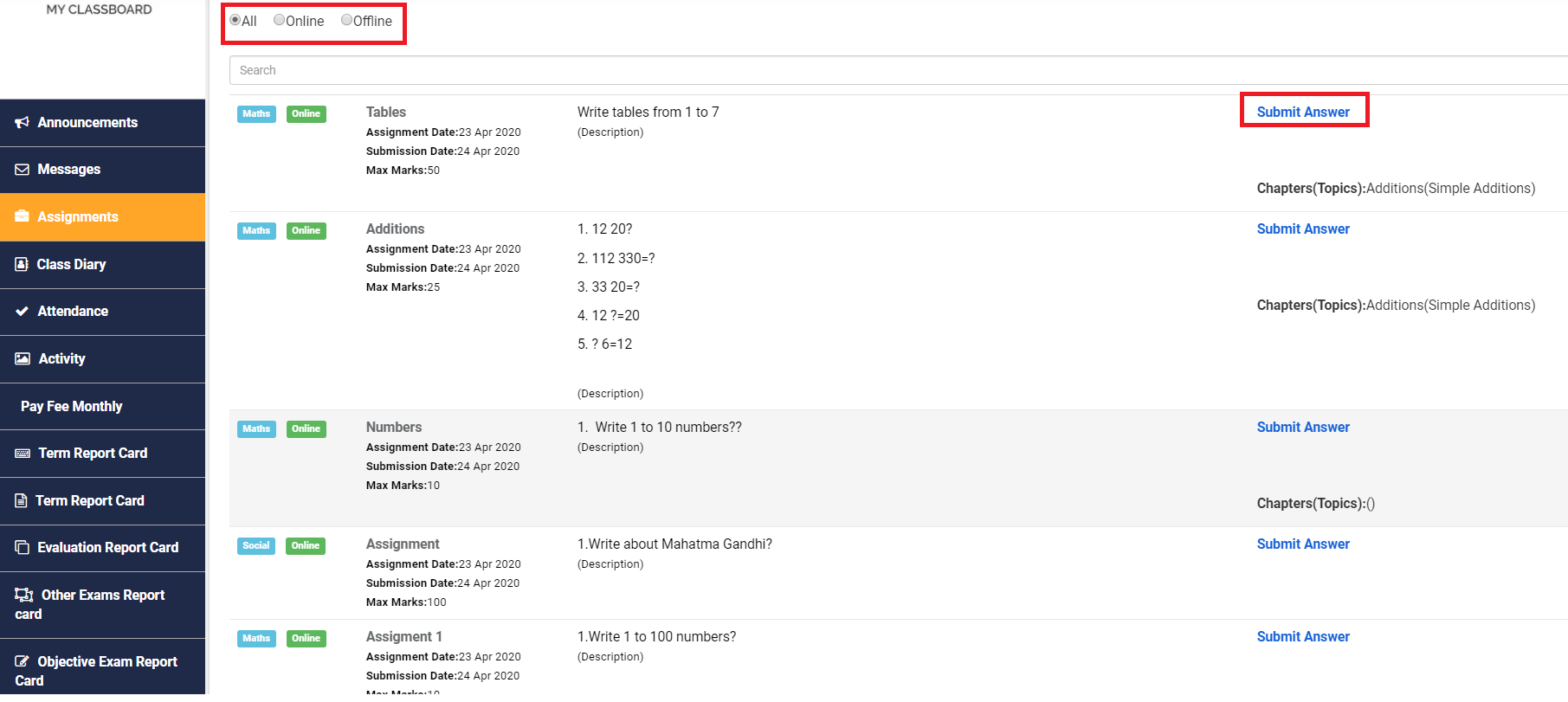This image features a digital interface of a platform named "My Class Board," which is designed for managing class assignments. Predominantly set against a white background, the interface includes a set of vertical menu options on the left-hand side, each accompanied by corresponding icons. These menu options listed from top to bottom are: Announcements, Messages, Assignments, Class Diary, Attendance, Activity, Pay Fee Monthly, Term Report Card, Another Term Report Card, Evaluation Report Card, Other Exams Report Card, and Object from Report Card.

Prominent on the screen is a blue bar situated to the left that changes to yellow when highlighted. Additionally, a red-circled rectangle appears at the top of the interface, presenting options labeled as "All," "Offline," and "Online." This selection seemingly allows users to filter content based on these categories.

In the main content area, assignments are listed and seem to be categorized by themes such as Tables, Additives, and Numbers. One particular assignment, titled "Submit Answer," is accentuated with a red box, indicating perhaps an immediate action or focus area. This detailed visual organization supports users in navigating and managing their educational tasks efficiently.